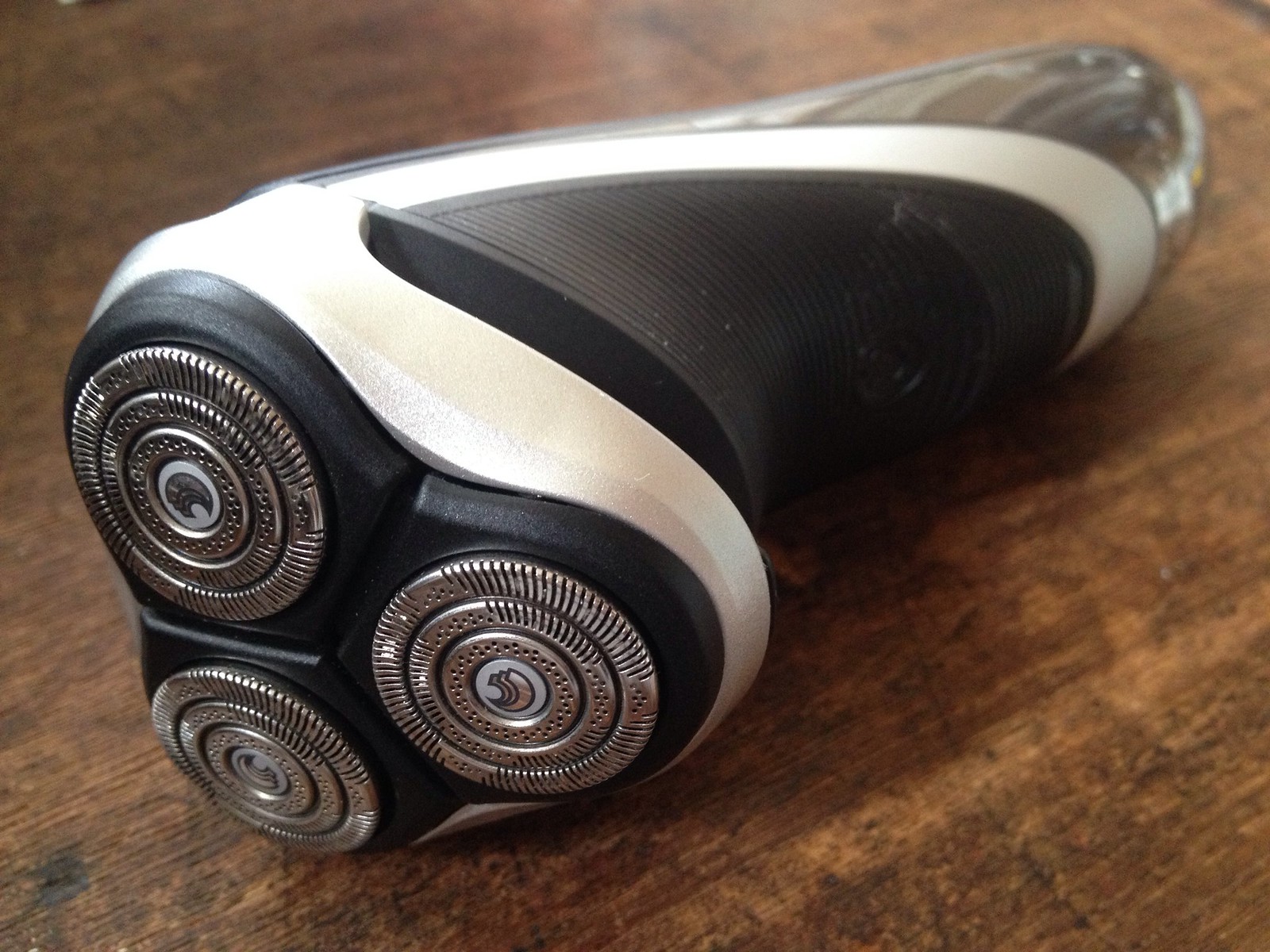This image features an electric shaver resting on a flat wooden surface, showcasing detailed grain and age marks of the brown wood. The shaver, primarily white and black in color, has a striking design with a triangular column at the top, where we observe three swirly, circular, metallic blades. Each blade is composed of three concentric circles. These blades are encircled by black plastic and set upon a silver background, contrasting with the textured horizontal lines on the front of the shaver. The cutting end of the machine points toward the bottom left corner, emphasizing the precision and design of the three secured cutting blades.